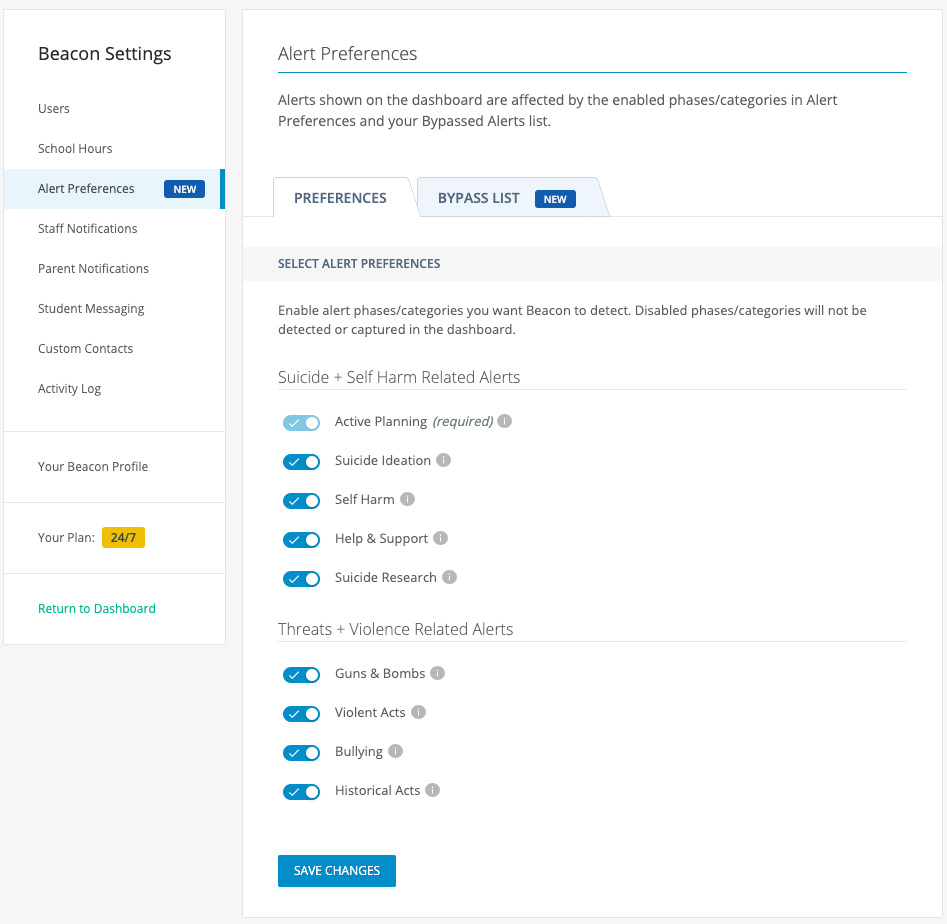The image appears to be a web page interface for a mental health and safety notification system designed for schools. On the left-hand side, there is a vertical menu with the following headings in order:

1. **Beacon Settings** 
2. **Users**
3. **School Hours**
4. **Alert Preferences**
5. **Staff Notifications**
6. **Parent Notifications**
7. **Student Messaging**
8. **Custom Contacts**
9. **Activity Log**

Below these headings, there is a box labeled **Your Beacon Profile** with options to **Enter Plan** and **Return to Dashboard**.

The central portion of the screen focuses on **Alert Preferences**, indicating that the alerts shown on the dashboard are influenced by the enabled phases, categories, alert preferences, and the user's bypassed alerts list. There are two tabs available: **Preferences** and **Bypassed List**.

Under the **Select Your Alert Preferences** section, there are categories aimed at possibly educators or administrators to monitor and respond to various student issues:

1. **Belongness (Suicide + Self-harm related alerts)**
   - Active Planning
   - Suicide Ideation
   - Self-harm
   - Help and Support
   - Suicide Research

Each of the above has a corresponding radio button to toggle the alert status as active or non-active.

2. **Threats and Violence related alerts**
   - Guns and Bombs
   - Violent Acts
   - Bullying
   - Historical Acts

This section also features radio buttons for activation and deactivation. At the bottom of this section, there is a prominent blue button labeled **Save Changes** to apply any adjustments made to the alert settings. 

Overall, this interface seems to be a comprehensive tool for school staff to manage and monitor alerts related to student mental health and safety effectively.